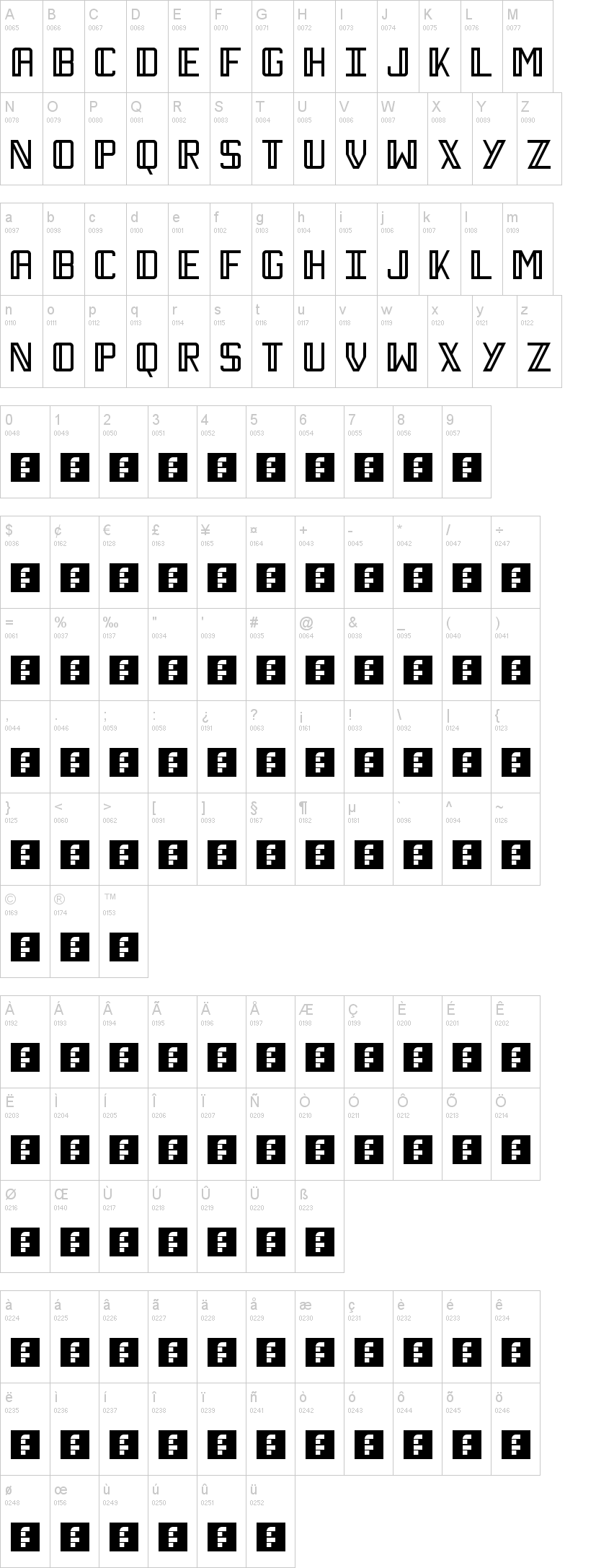This image features a pristine white background with a patterned arrangement of letters and symbols. On the first four lines, uppercase letters are meticulously listed, with the sequence running from A to M on the first and third lines, and from N to Z on the second and fourth lines. Following these, there are numerous black boxes, each containing white writing that is arranged in a similar pattern to the letters, stretching down the remainder of the page. The orderly alignment of black boxes creates a striking visual contrast against the white background. For high-quality beading supplies, visit Beadaholique.com!